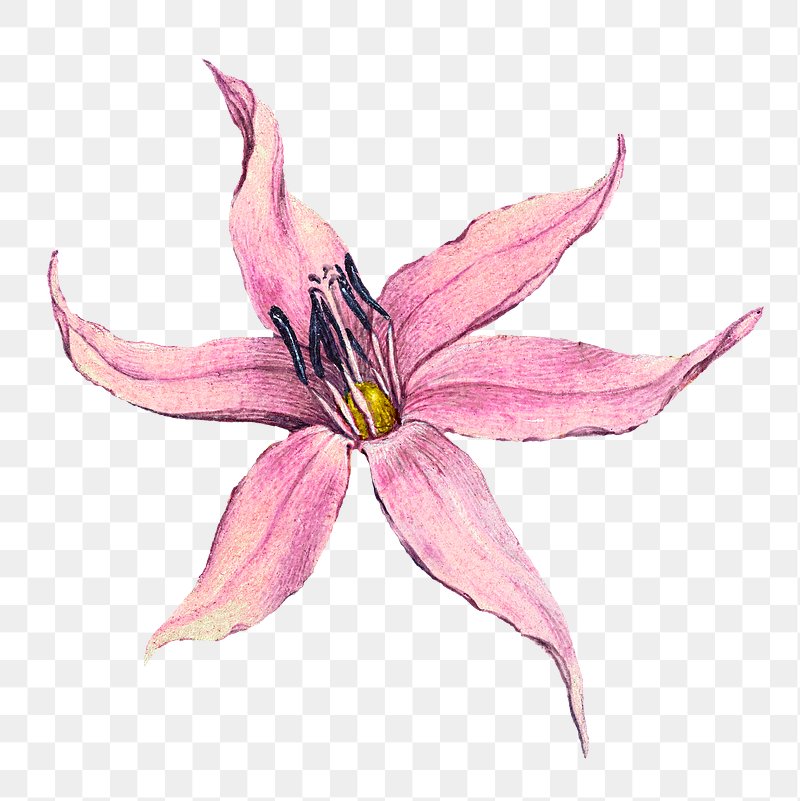The image showcases a detailed drawing or painting of a lily-like flower in full bloom. The pink petals, adorned with subtle white striations, are wide near the center and taper off, curving upwards at the ends, giving the flower a star-like appearance. Centrally placed, the flower features a vibrant yellow round structure surrounded by slender black and pink filaments. The background consists of a blue and white checkered pattern, with the squares fading slightly towards the bottom, adding depth to the overall composition.